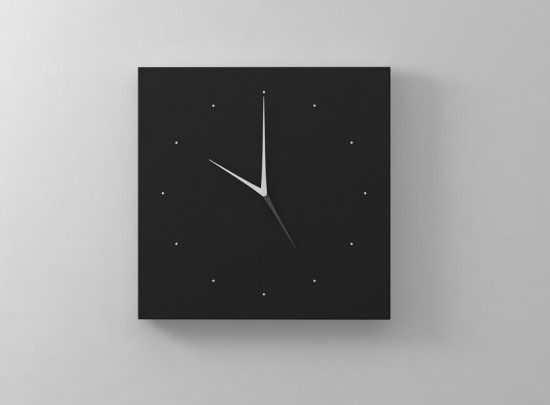A square black clock is centered against a predominantly white background, with a light source illuminating from the top left. The bottom right corner of the background transitions into a mostly gray shade. The clock has a modern design with a black clock face and 12 equally spaced dots representing the hours, arranged in a circular pattern. The white hour hand is pointing at 10, the white minute hand is positioned at 12, and the dark second hand is indicating 5.